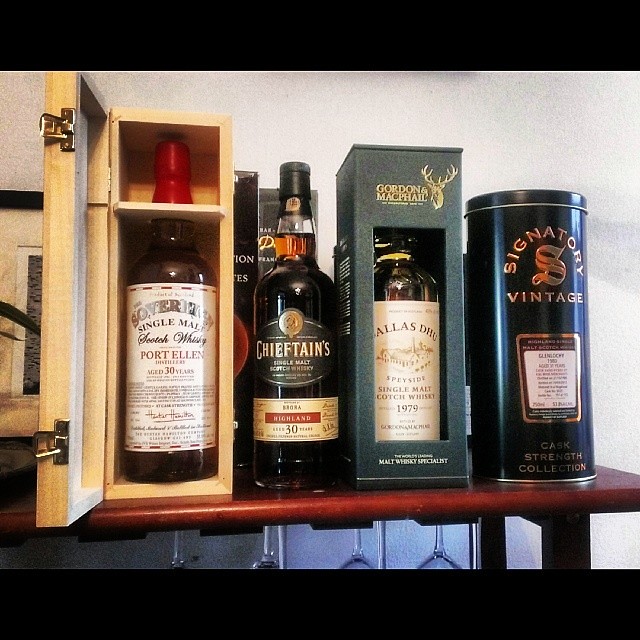The photograph captures an indoor setting with a horizontally rectangular frame, bordered by black strips at the top and bottom, featuring a brown-toned wooden shelf adorned with upscale liquor bottles and wine glasses hung upside down from its underside. Displayed prominently on the shelf are four meticulously arranged high-end single malt Scotch whiskeys, a clear indication of their collector's item status.

From left to right: the first offering is nestled in an open wooden box and identified as a glass of Port Ellen Distillery's Sovereign Single Malt Scotch Whiskey, aged 30 years. Adjacent to it stands a solitary bottle of Chieftain's Single Malt Scotch Whiskey from Highland, also aged 30 years, strikingly black and elegant in its simplicity. The third item is ensconced in a gray box with a transparent cellophane front, revealing a bottle with the Gordon and McPhail label and an emblem of a large buck; it is a single malt Scotch whiskey bottled in 1979. The final bottle, housed within a cylindrical aluminum container, belongs to the Signatory Vintage Highland Single Malt Scotch Whiskey collection, part of the Cask Strength Collection, and indicates a bottling year of 1980.

The overall image is characterized by its high clarity and quality, accentuated by the natural light that enhances the detail and presentation of the prized whiskey collection on display.